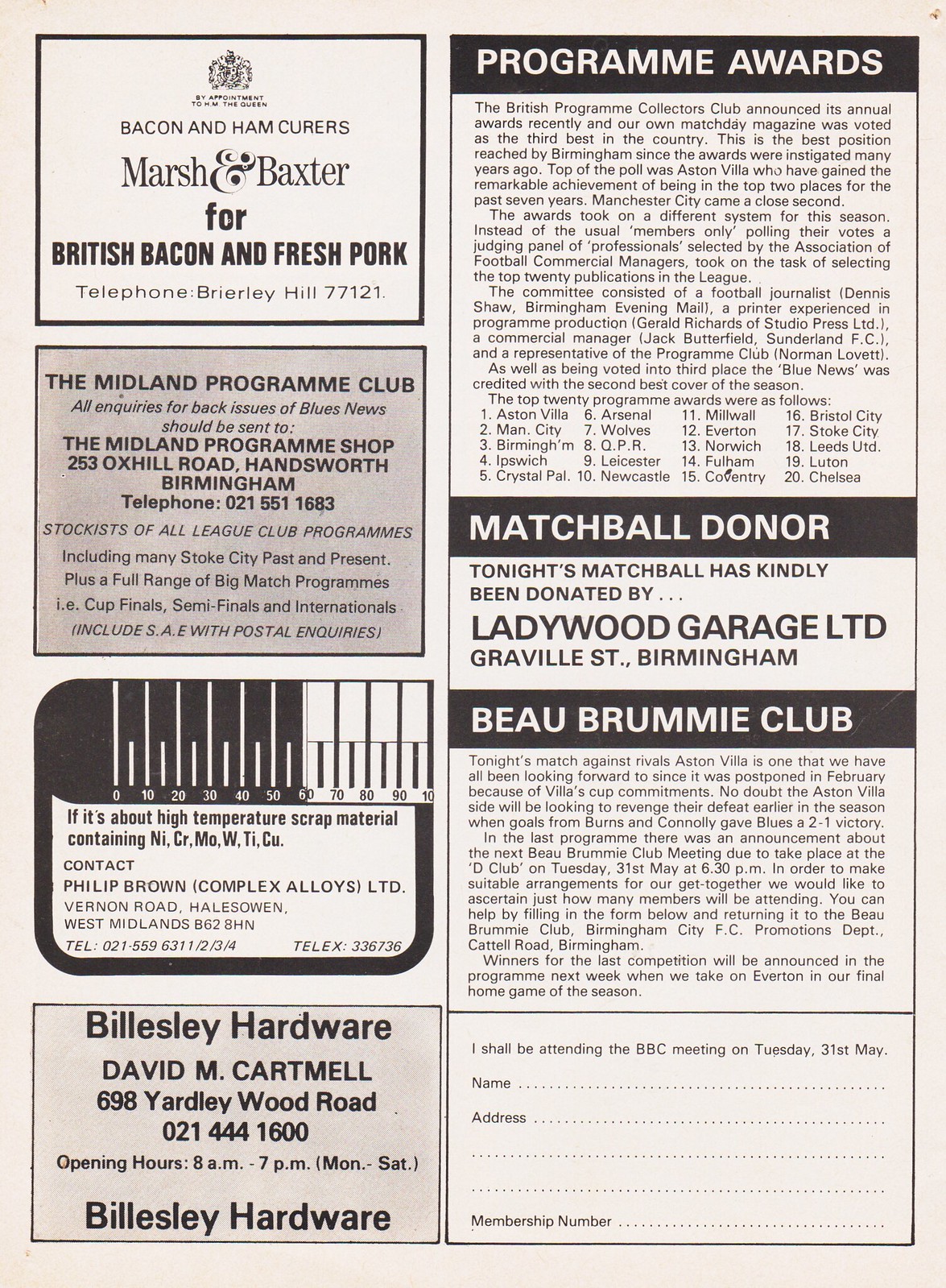This black and white page from a magazine or program features a series of rectangular sections, each containing either an advertisement or an article. The top left advertisement is for Marsh and Baxter, promoting British bacon and fresh pork, with contact information for Burke Burley Hill. Underneath is an ad for the Midland Program Club, detailing its location in Birmingham and its contact number. The following advertisement mentions high-temperature scrap metal materials from Philip Brown Complex Alloys LTD. At the bottom of this column, there is an ad for Billis Lee Hardware, managed by David M. Cartmill, with its store hours listed.

On the right side of the page, the top section discusses match ball donor awards, noting that tonight’s match ball has been kindly donated by Ladywood Garage LTD from Gravel Street, Birmingham. Below this, there is a small fill-out card, stating, "I will be attending the BBC meeting on Tuesday, 31st of May," and requesting the attendee’s name, address, and membership number. Finally, the bottom right of the page features an article about British Soccer, hinting that the entire publication may be dedicated to English football, with relevant advertisements and information.